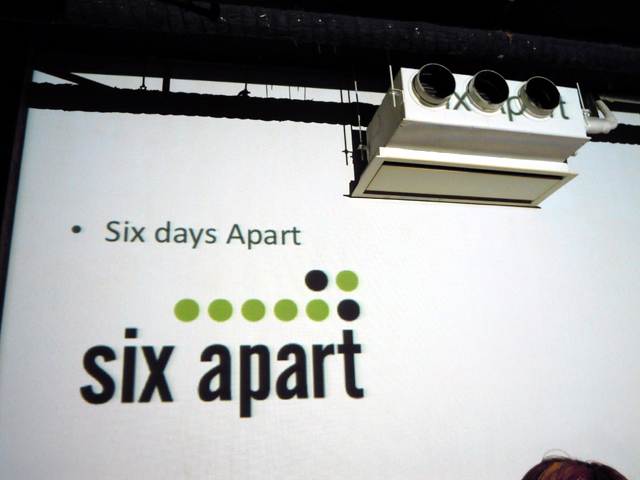A detailed photograph capturing a presentation projected onto a large white screen. The slide prominently features the phrases "six days apart" and, in larger bold letters, "six apart". Below these texts, there are two rows of dots: the top row contains two dots while the bottom row consists of six dots. In the top row, the first dot is blue (or dark green), and in the bottom row, the sixth dot is blue (or black), with the remaining dots in varying shades of green or lime green. The white screen dominates the image, but in the top right corner, there is a noticeable rectangular metal structure with three circular projections attached to the ceiling. Additionally, the top of a spectator's head with light brown hair is visible in the bottom right corner of the image. The photograph communicates a sense of some clever or meaningful coding represented by the colored dots and their arrangement.